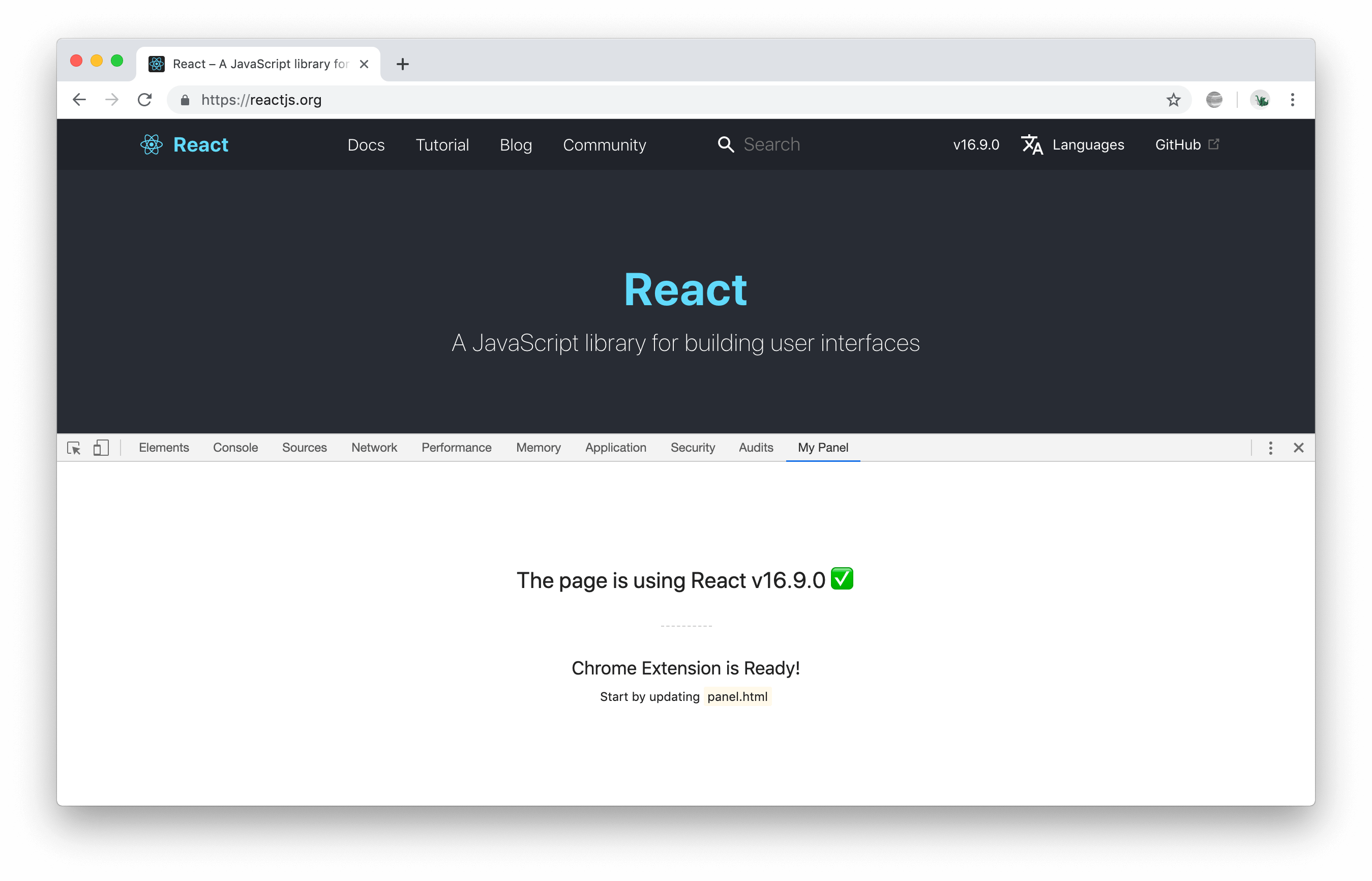A detailed caption for the described image could be:

"This screenshot displays a webpage viewed in a web browser. In the top-left corner of the browser window are the customary red, yellow, and green circles used for window controls on a Mac, positioned next to the first browser tab. The tab's title begins with 'React, a JavaScript library for' but is truncated. Adjacent to this tab is an 'X' to close it, and a '+' symbol for opening a new tab. The browser toolbar contains navigation buttons, including a back arrow, forward arrow, refresh icon, and a lock symbol, indicating a secure connection with 'HTTPS://reactjs.org.' Further right are buttons for accessing favorites and user profile settings.

Centered on the webpage is a prominent logo of an atom depicted in blue, representing React. Underneath this logo are navigation links labeled 'Docs,' 'Tutorial,' 'Blog,' and 'Community.' To the right of these links is a search icon accompanied by a search bar. Just below this bar, the version number 'v16.9.0' is indicated, followed by links for different languages and a GitHub repository.

The main content area displays the text: 'React - A JavaScript library for building user interfaces.' Below this, various browser tabs are open, including 'Elements,' 'Console,' 'Sources,' 'Network,' 'Performance,' 'Memory,' 'Application,' 'Security,' 'Audit,' and 'My Panel.' A message at the bottom confirms that 'This page is using React v16.9.0' with a green checkmark verifying correctness. Additionally, a tooltip in the corner notes that the 'Chrome extension is ready,' advising users to 'Start by updating panel.html.'"